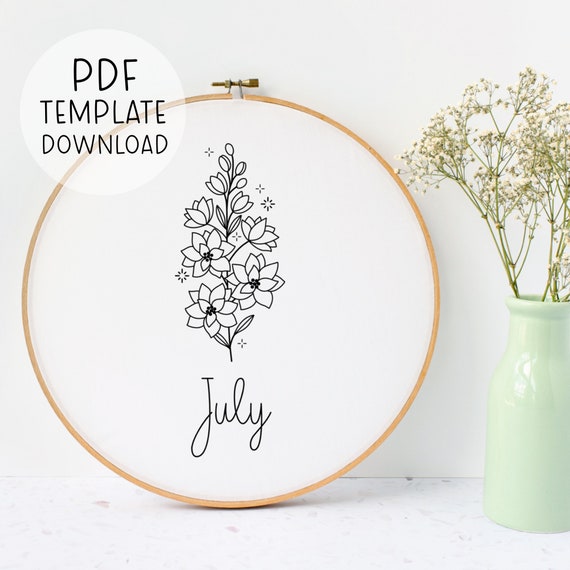An indoor, well-lit photograph showcases a beautifully styled scene ideal for a website promoting a downloadable PDF template. The photo features a white-walled background adorned with a large, circular bamboo embroidery hoop at its center. Inside this hoop, a white fabric is stretched tightly, displaying a simple black outline drawing of flowers on a stem, with the word "July" elegantly scripted beneath the motif. To the right of the embroidery hoop stands a celadon green vase, reminiscent of an old milk bottle, filled with delicate stems of baby's breath flowers. In the upper left corner of the image, a translucent white circle serves as a watermark, inscribed with the text "PDF template download," subtly promoting the downloadable content.